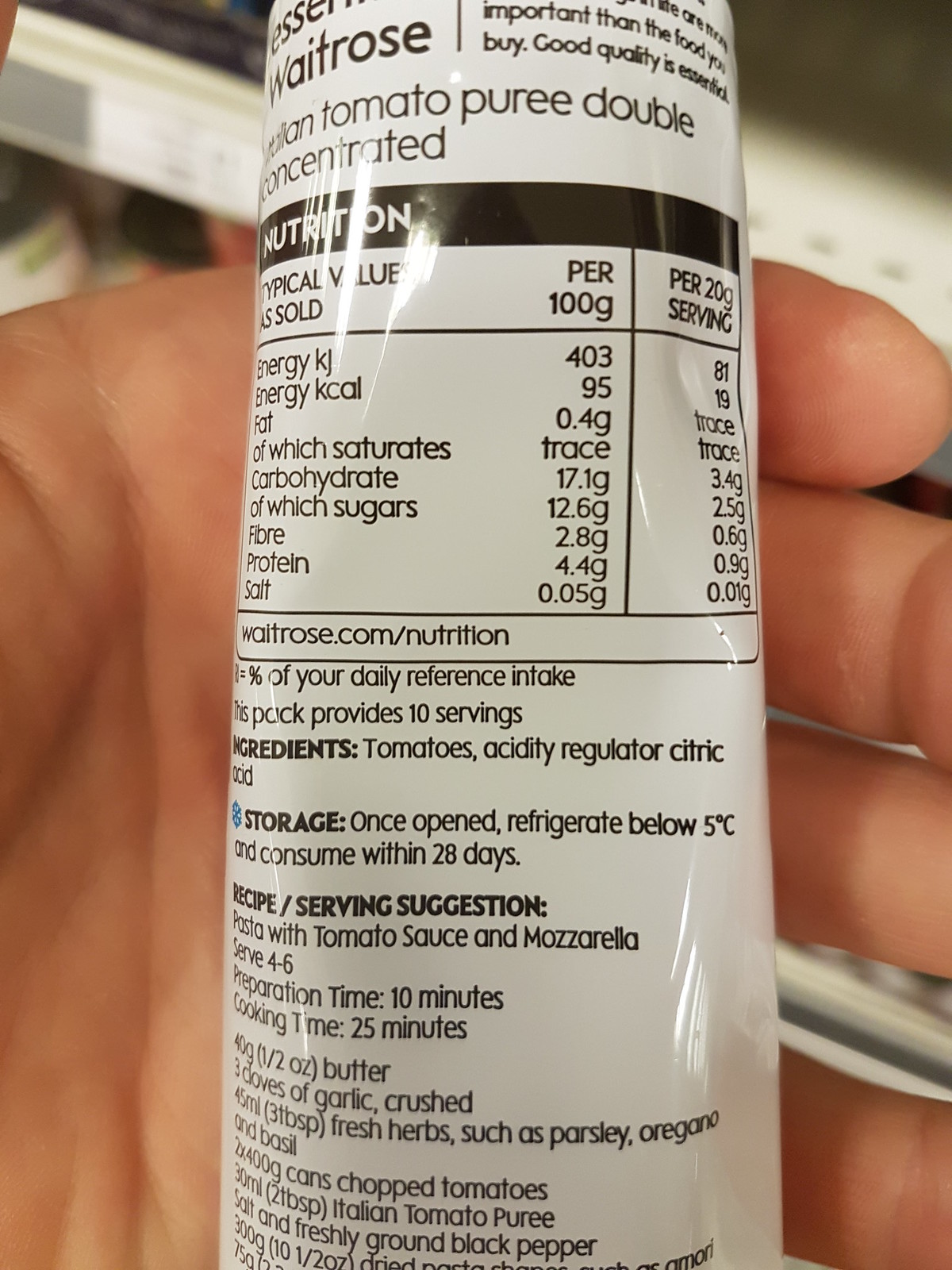This image showcases a white tube, likely containing tomato paste, adorned with black text. Key details inscribed on the packaging include various recipes and serving suggestions, highlighted by a dish of pasta with tomato sauce and mozzarella, which serves 4-6 people and has a preparation time of 10 minutes, with a total cleaning time of 25 minutes. The label also instructs that, once opened, the product should be refrigerated at a temperature below 5 degrees Celsius and consumed within 28 days. Above these instructions is a list of ingredients, including tomatoes and acidity regulators such as acidic acid. The packaging notes that the tube provides approximately 10 servings.